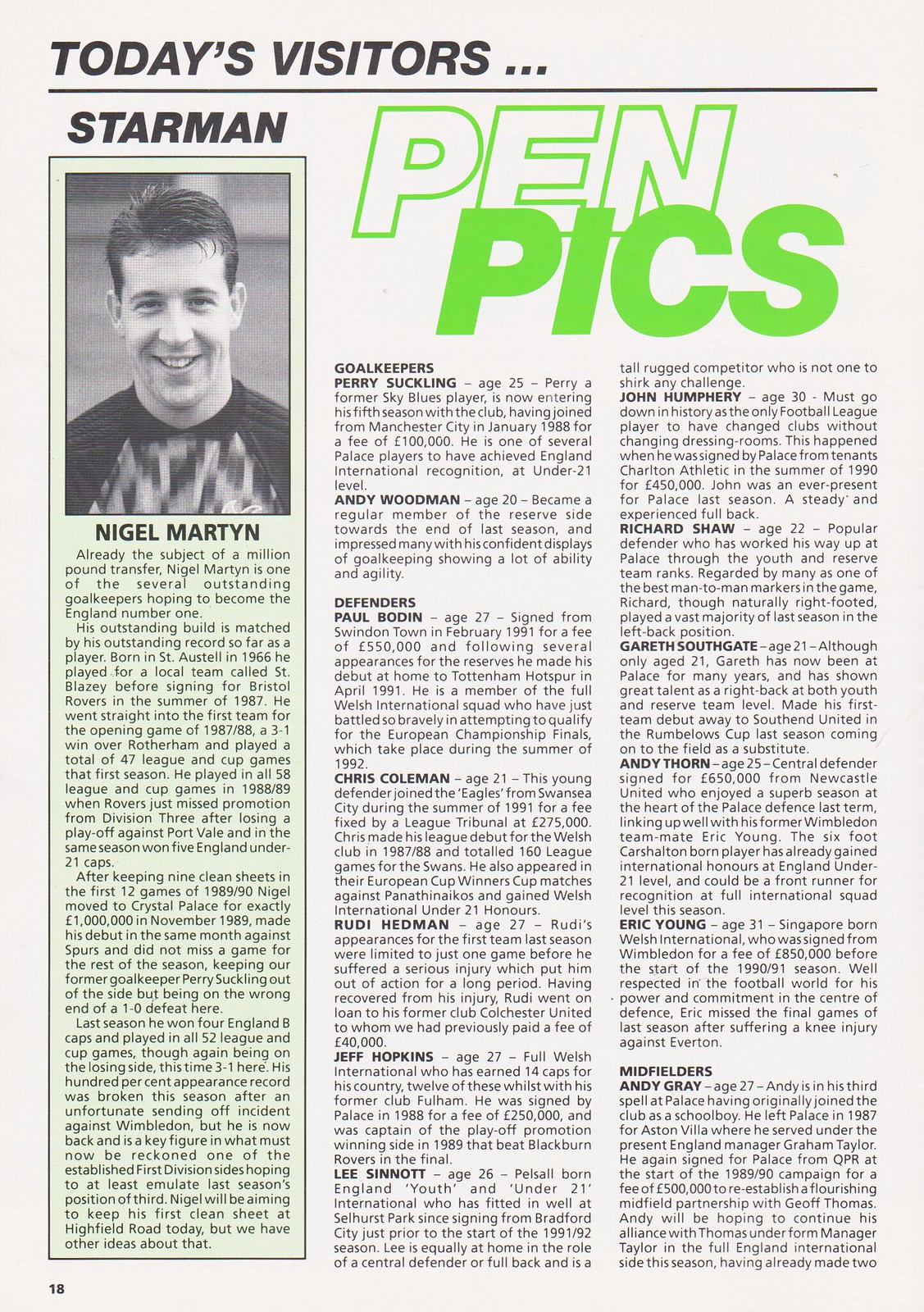The image is a detailed page taken from a sports magazine, sporting the header "Today's Visitors" at the top, underlined for emphasis. The left side of the page features a bold section titled "Starmen," accompanied by the image of a young man in a soccer jersey identified as Nigel Martyn. Below his photo, Nigel Martyn's name is displayed, and the section includes three paragraphs elaborating on him, tinted in a light green hue.

On the right side of the page, there are two columns under the heading "Pin Picks" written in green font. This part of the page lists various players alongside their positions and ages. Among those listed under goalkeepers are Perry Suckling, age 25, and Andy Woodman, age 20. Under defenders, we find Paul Bowden, age 27, Chris Coleman, age 21, Rudy Hedman, age 27, Jeff Hopkins, age 27, Lee Sinat, age 26, and John Humphrey, age 30. A single midfielder is also mentioned. This comprehensive article about Nigel Martyn, renowned as a leading goalkeeper in England, is found on page 18 of the publication, and it notes that the featured athletes are generally in their early to late 20s.